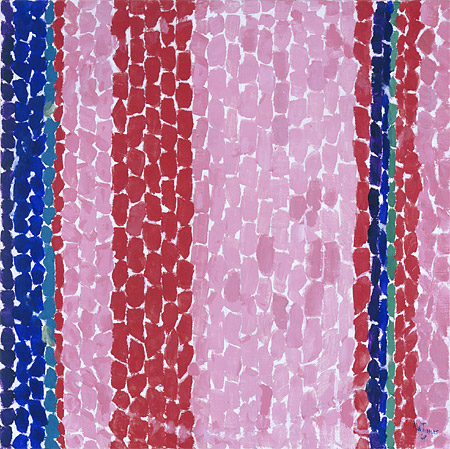The image is an abstract artwork, possibly a painting, featuring a complex assemblage of vertical stripes made up of stone-like shapes. The background is predominantly a variety of blues, reds, and pinks, with each color forming its own vertical stripe. Starting from the left, there is a thin band of dark blue, almost black, followed by two bands of royal blue, then a single stripe of aquamarine blue. Next is a vertical stripe of red, followed by three slightly wider stripes of pink stones. The sequence continues with five red stripes, leading into a central section that consists of about ten strands of various shades of pink with occasional white gaps between them.

Further to the right, the pattern includes a single strand of red stones, another single strand of dark blue, a strand of lighter blue, followed by two stripes of red, and finally two more strands of lighter pink stones with white gaps interspersed. The stones-alike shapes stacked vertically give the impression that the lines are slightly irregular and fragmented. The most striking elements are the central pink mottling, surrounded by these varied blues and reds, creating a visually engaging and dynamic composition.